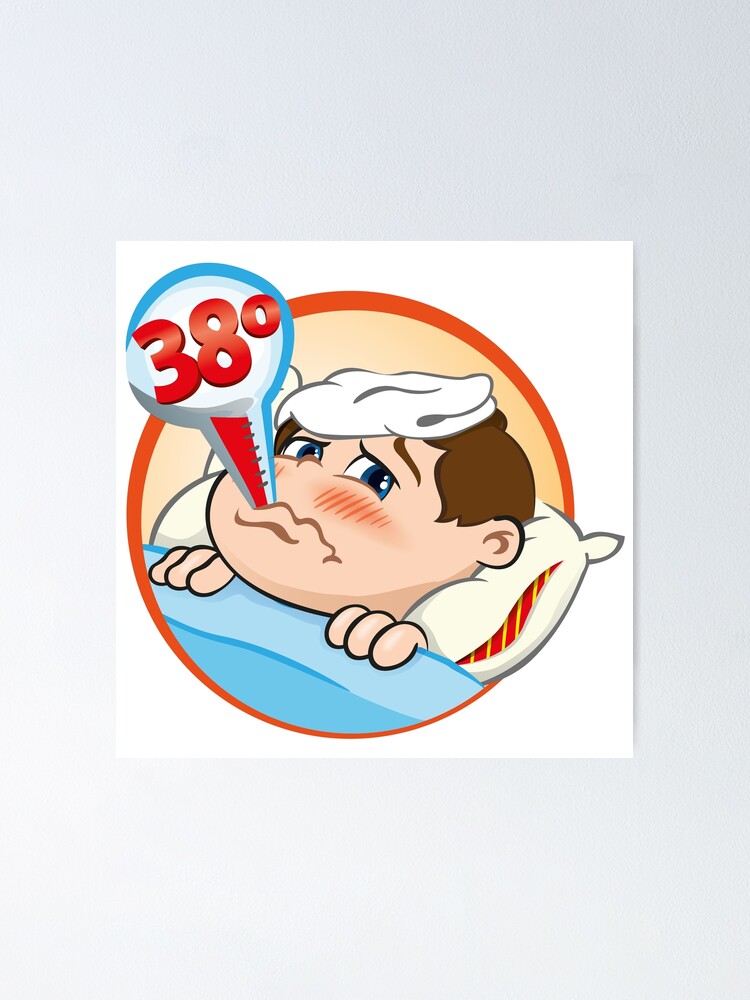The rectangular image, taller than it is wide, features a gray background with a centered white square. Inside the white square is an orange circle with a cream-colored inner section that contains a detailed cartoon drawing. The cartoon depicts a young boy with brown hair, big blue eyes that appear teary and sad, and rosy red cheeks, indicating he has a fever. A white washcloth or cold compress rests on his forehead. The boy is lying on a white pillow that has red and yellow stripes on the inner part. He holds a blue bedsheet or comforter with just his fingers visible. Emerging from his mouth is a thermometer, colored white, blue, and red, displaying a temperature of 38 degrees.